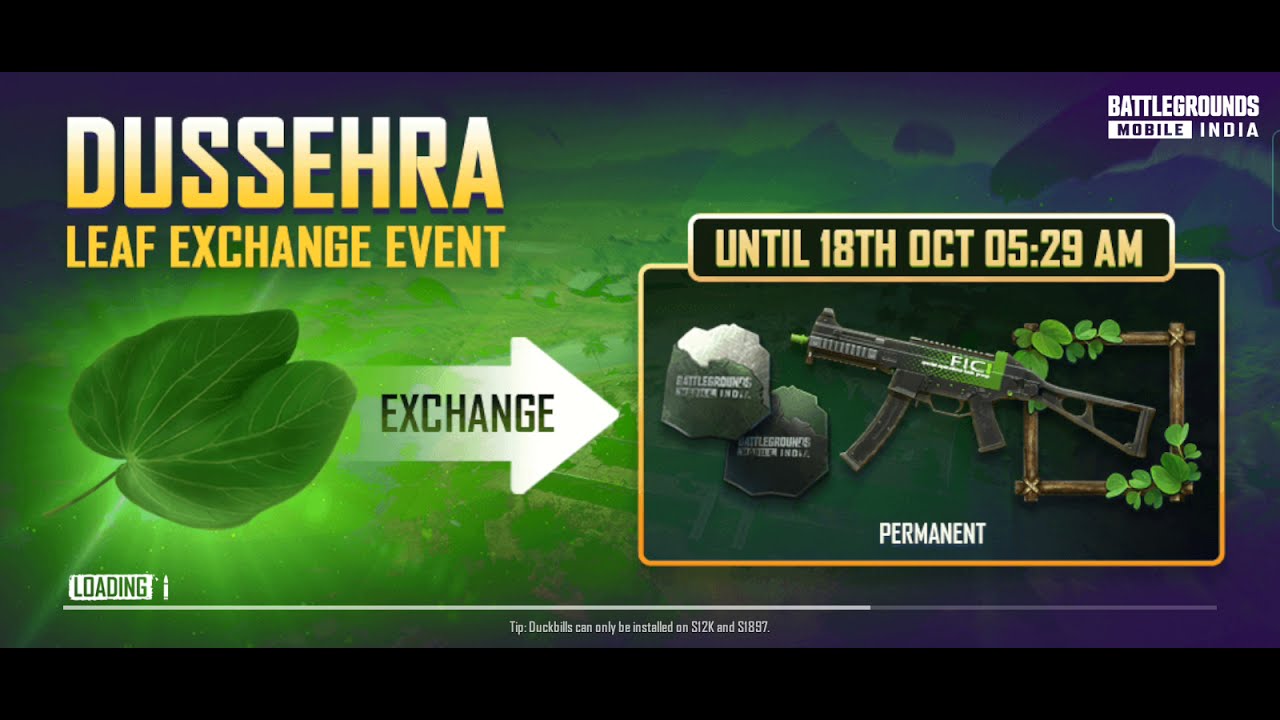The image showcases a promotional screen from the video game Battlegrounds Mobile India, centered around a special Dussehra Leaf Exchange event. Dominating the image is a green leaf emitting vibrant, glowing green rays, accompanied by a white arrow labeled "exchange," pointing towards a gold-trimmed box. The text above reads "Dussehra Leaf Exchange Event," highlighting the event. In the top right corner, "Battlegrounds Mobile India" is clearly visible. Below, the image displays a machine gun with distinct green detailing on its body and tip, positioned next to a wooden crate adorned with green leaves. The date and time "until 18th October 05:29 a.m." is indicated above the rifle. The overall aesthetic is marked by green and yellow hues reminiscent of St. Patrick's Day, with silver accents. Additionally, there are small tags with the word "Battlegrounds" and a note at the bottom indicating that "tip duck bills can only be installed on S12K and S1897" shotguns, noting specific in-game mechanics. The image is approximately 75% loaded, hinting at an engaging new update or feature for the game.